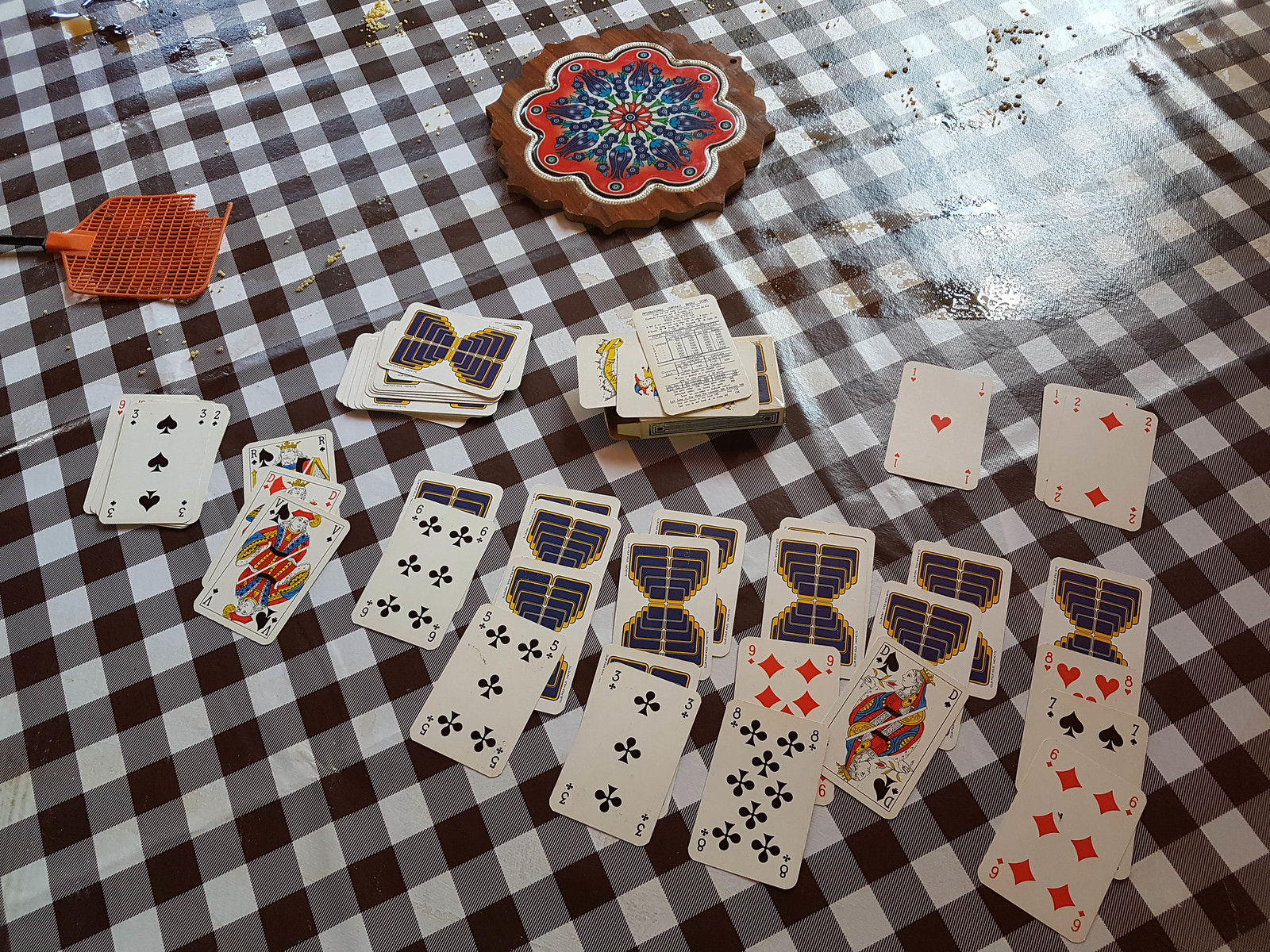This indoor color photograph captures a slightly angled, overhead view of a tabletop covered with a white and dark gray checkered tablecloth. The lower half of the image is dominated by a spread of playing cards, organized in eight rows, suggesting a game of solitaire in progress. These cards are primarily oriented vertically, though they overlap each other in an untidy manner. 

Beginning from the left, the first row shows the Three of Clubs. To its right, a stack starting with the King of Spades, topped by the Queen of Diamonds and the Jack of Spades. Next, the Six of Clubs is seen, followed by the Five of Clubs, and another Three of Clubs. The second row features the Nine of Diamonds next to the Eight of Clubs. Following these, the Queen of Spades appears, alongside the Eight of Hearts, Seven of Spades, and the Six of Diamonds. Some cards in the rows are facedown, displaying a blue and yellow pattern.

To the right of the image's center, the Ace of Hearts and Two of Diamonds are visible. In the very middle, the open card box, displaying Jokers and instructions, is clearly noticeable. 

In the upper left corner, part of a blue fly swatter with a broken edge intrudes from the side. At the top center, a wooden pot holder or trivet adorned with a blue and red floral design sits near the edge of the table. 

Scattered debris, food stains, and water or soda droplets are visible on the tablecloth, adding a touch of realism to the scene.